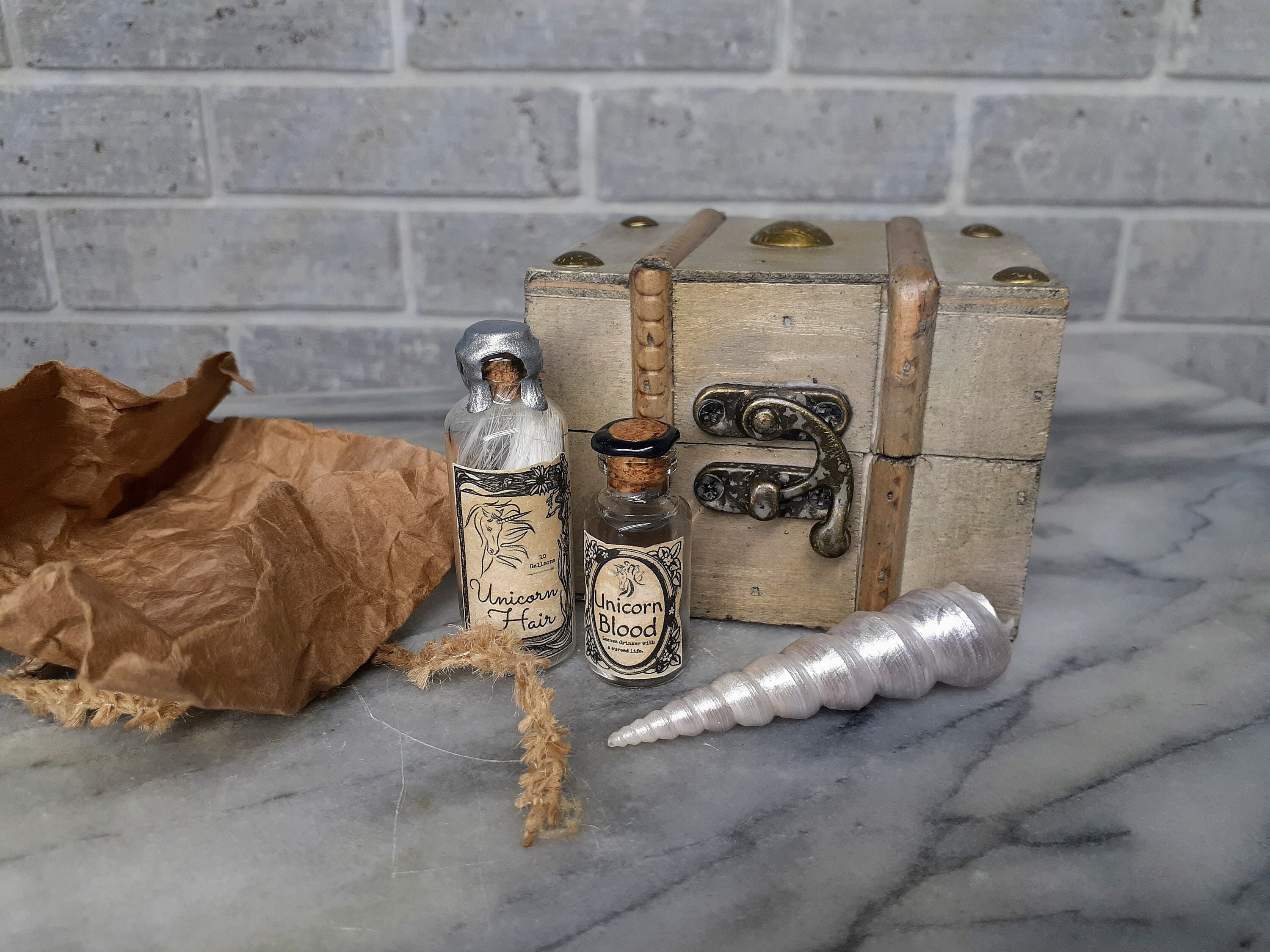The photograph showcases an artfully arranged collection of mystical-themed objects displayed on a marble table against a gray brick wall. Central to the composition is a small, pirate chest-like wooden box with weathered brass hardware—specifically, four corner brackets and a prominent circular metal plate in the middle, alongside a rusty black-painted latch handle. Surrounding the box are two glass apothecary bottles: one labeled "Unicorn Blood," which has a brown cork and appears designed to hold liquid, and the other, a taller bottle labeled "Unicorn Hair," featuring wisps of white hair and sealed with silver wax. In front of the box lies a silvery, spiral-shaped item resembling a unicorn horn. To the left, a crumpled brown paper bag with frayed strands of rope adds rustic charm to the composition. The entire scene suggests an old-timey apothecary kit, steeped in fantasy elements.